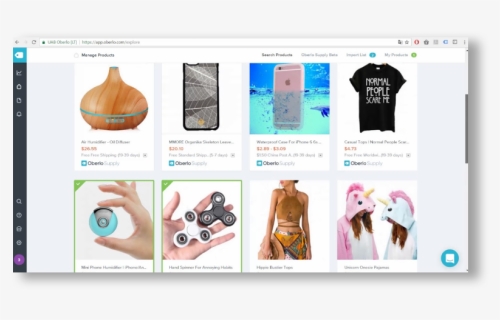This image is a low-resolution screenshot captured from a web browser, evident from the visible browser icons at the top. The screenshot depicts a section of a shopping website featuring a grid layout with four square white blocks arranged in two rows. Each block contains an image and accompanying text, both of which are challenging to discern due to the low quality of the image. These blocks represent clickable product links showcasing a variety of items for sale. The assortment of products is eclectic, lacking a common theme, and includes items such as an oil diffuser, a phone case, a t-shirt, a fidget spinner, various clothing pieces, and a character onesie. The text within each block is unfortunately too small to be legible, further hampering the ability to identify the finer details of each product.